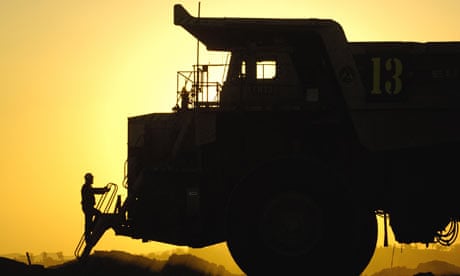The photograph captures a striking yellow sunset with accents of orange framing the scene, creating a vibrant backdrop that casts the entire foreground in black silhouette. Dominating the right side of the image is an industrial-size dump truck, its massive wheels, rear bucket, and small square window clearly outlined against the glowing sky. In front of the truck, a man's silhouette is seen climbing a ladder or wire steps leading to the front engine area, though his exact actions remain unclear. The base of the photograph reveals an uneven, wavy land mass also silhouetted by the vivid sunset, adding texture to the scene. This powerful image contrasts the large tractor and the man with the wide expanse of glowing sky, emphasizing the rugged landscape and industrial elements.